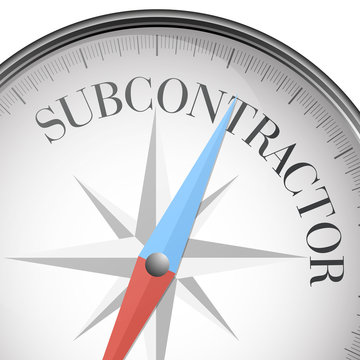This digital image appears to be a stylized drawing of a compass, likely created as clip art or a logo for a presentation or website. The compass is prominently featured, occupying most of the space but slightly hugging the bottom part of the image. The compass lacks traditional directional points and instead displays the word "SUBCONTRACTOR" in large, black, uppercase letters inside the compass. The border of the compass is gray and black, with various line markings similar to those on a clock face—some thicker and darker, and some shorter and lighter. The interior of the compass is white, and in the center, a needle is fastened with a round nail. The needle itself is divided into two colors: blue and red, with additional smaller, gray needles positioned behind it. A star shape, rendered in dark and light gray, forms the backdrop within the compass, giving the appearance of a classic compass design. The blue part of the needle is pointing upwards, adding to the navigational theme of the image.